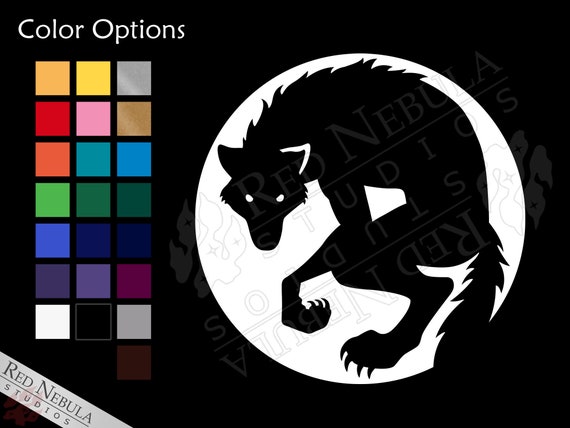The image appears to be a screenshot from a digital image creator associated with Red Nebula Studios, as indicated by the faint watermark and logo in the bottom left corner. The background is predominantly black, accented with a prominent white circle in the center showcasing a silhouette of a black werewolf with beady white eyes. The werewolf's silhouette is detailed, featuring drawn-up claws on one hand and a bushy tail. To the left side of the image, the words "color options" are displayed in white, followed by three columns of color selection squares. These squares offer a wide range of colors, including various shades of yellow, gray, pink, blue, green, purple, black, white, orange, and brown. The overall layout is reminiscent of a paint-by-numbers or customizable art tool, suggesting an interactive art creation environment.